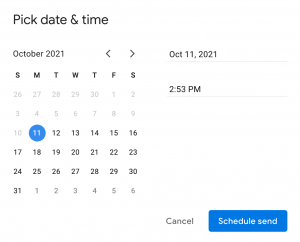The image depicts a computer screen displaying a calendar interface for scheduling purposes. The background of the interface is white, while the text is in black. At the top of the calendar, the phrase "Pick Date and Time" is prominently displayed. Directly below this, it shows "October 2021" with navigation arrows on either side, allowing the user to move to the previous or next month. The top row of the calendar layout is labeled with the initials of the days of the week: SMTWTFS (Sunday through Saturday). 

The specific date selected is October 11, 2021, marked distinctly by a blue circle around the number 11. Additionally, the time chosen is 2:53 PM. The calendar grid itself shows the transition from the previous month, with the last few days of September (26th to 30th) in a faint gray. The beginning of October (1st to 10th) is also in gray, indicating they are past dates. From October 12 onwards, the dates are in standard dark print, clearly visible, signifying upcoming dates. 

At the bottom right corner of the calendar interface, there is a "Schedule Send" button for finalizing the appointment or event.